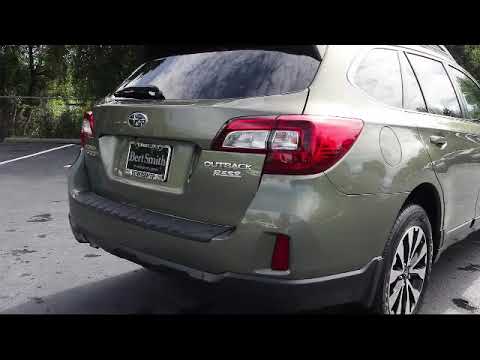A detailed photograph captures the back end of a dark olive green Subaru Outback parked diagonally in a blacktop parking lot. The image, framed by black bands at the top and bottom, shows the car's red taillights with a clear or white light in between. The car's license plate reads "Burt Smith" in gray letters on a black background, bordered by a silver frame. Positioned above the plate is the Subaru insignia, and “Outback” is emblazoned in silver letters accompanied by some smaller, indistinguishable text below. The Subaru features black tires with silver hubcaps and dark tinted windows. Visible in the background are green trees and a hint of grass, adding a natural contrast to the setting. The car’s surface reflects the surrounding environment, suggesting a sunny day, and the ground is marked with white parking stripes and black splotches.